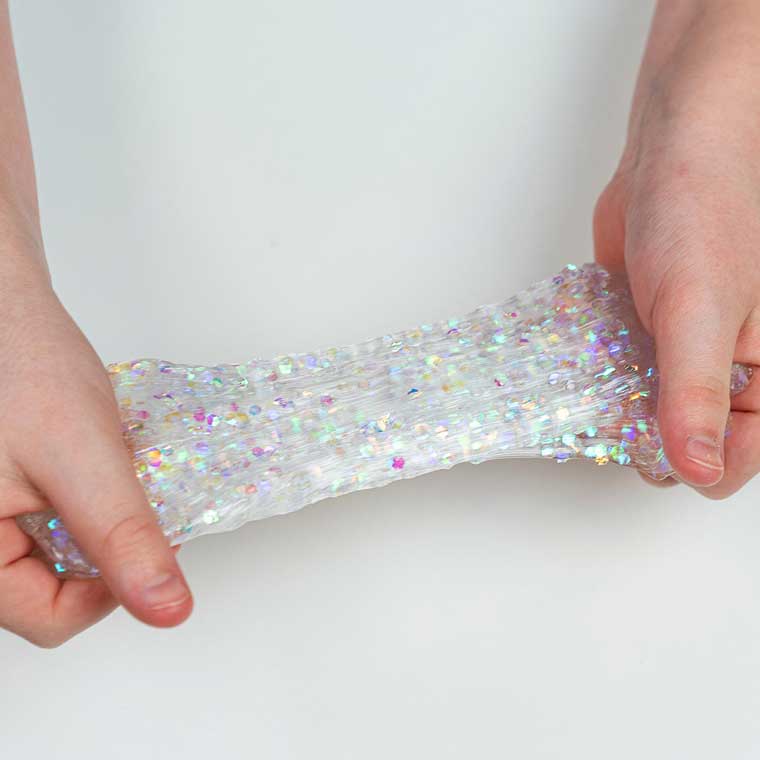In this captivating image, two hands, descending from the top of the frame, are seen pulling a clear, stretchy piece of plastic. The left hand extends slightly lower than the right. Each thumb rests atop the plastic while the partially visible index fingers curve underneath. The right hand is visible up to the wrist, whereas the left hand extends a bit further down. The plastic, transparent save for its colorful, shiny circular patterns in pink, blue, white, and yellow, is being stretched taut across the frame. The overall effect showcases the elasticity and vibrant design of the plastic.